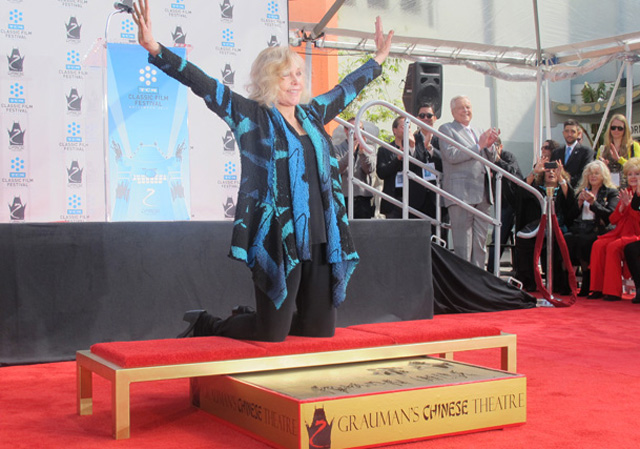The photograph, captured outdoors, features an older woman with slight graying hair kneeling on a gold bench with red seat cushions, in front of a section of wet cement, likely having just made her handprints and signed her name. She is dressed in black pants, a black shirt, and a blue and black cardigan. Behind her, on a raised stage, a poster reading "Classic Film Festival" is visible atop a wall. Further back to the right, a happy crowd is gathered, clapping, and taking pictures. Underneath the bench, the inscription "Grauman's Chinese Theatre" can be seen. The setting includes a red carpet and black stage with stairs and metal railings, accentuated by a red velvet rope. The woman appears joyful, with arms outstretched, as she celebrates this memorable moment.